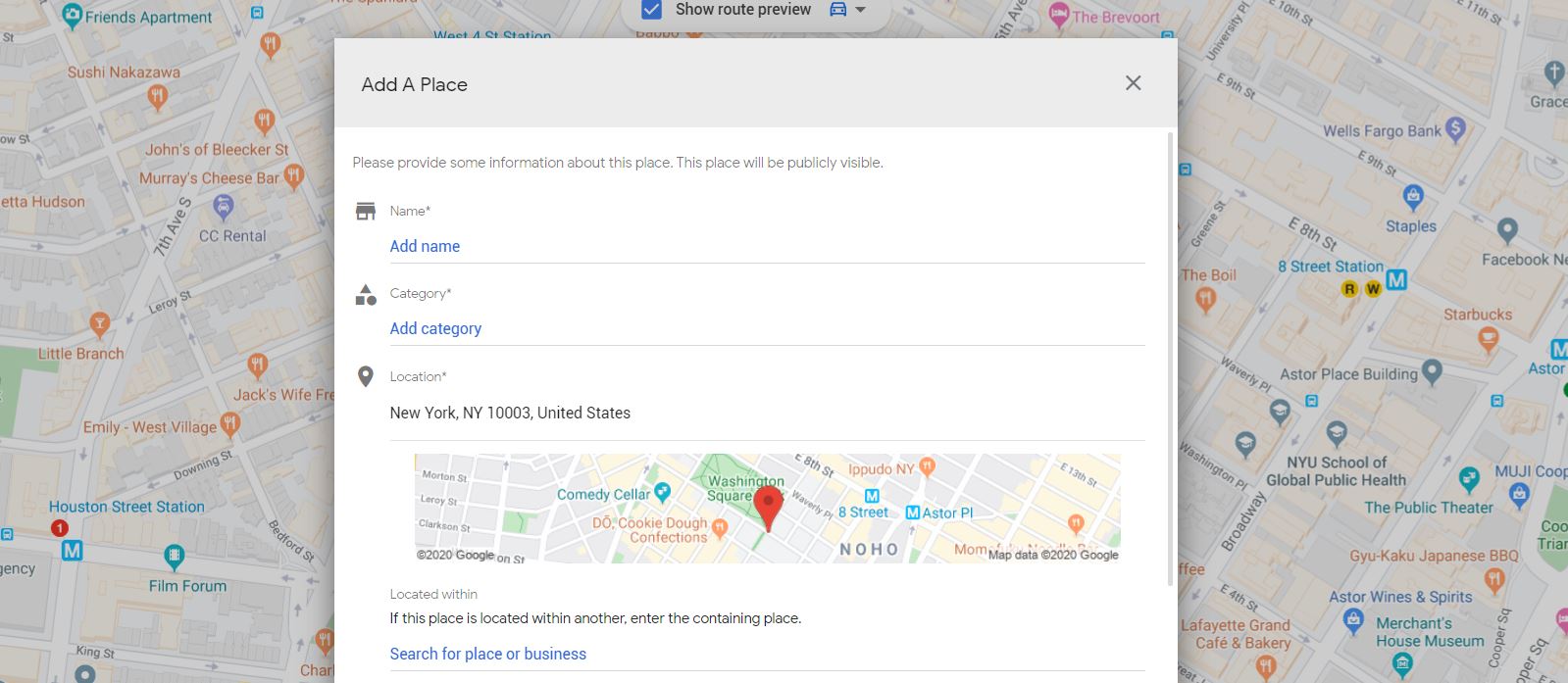This image is a screenshot from a navigation app displaying an unidentified city. Overlaying the map is a dialog box labeled "Add a Place." In this menu, users are instructed to provide a name, select a category, and specify a location for the place to be added. The location is marked by placing a red pin on the desired spot within the city map.